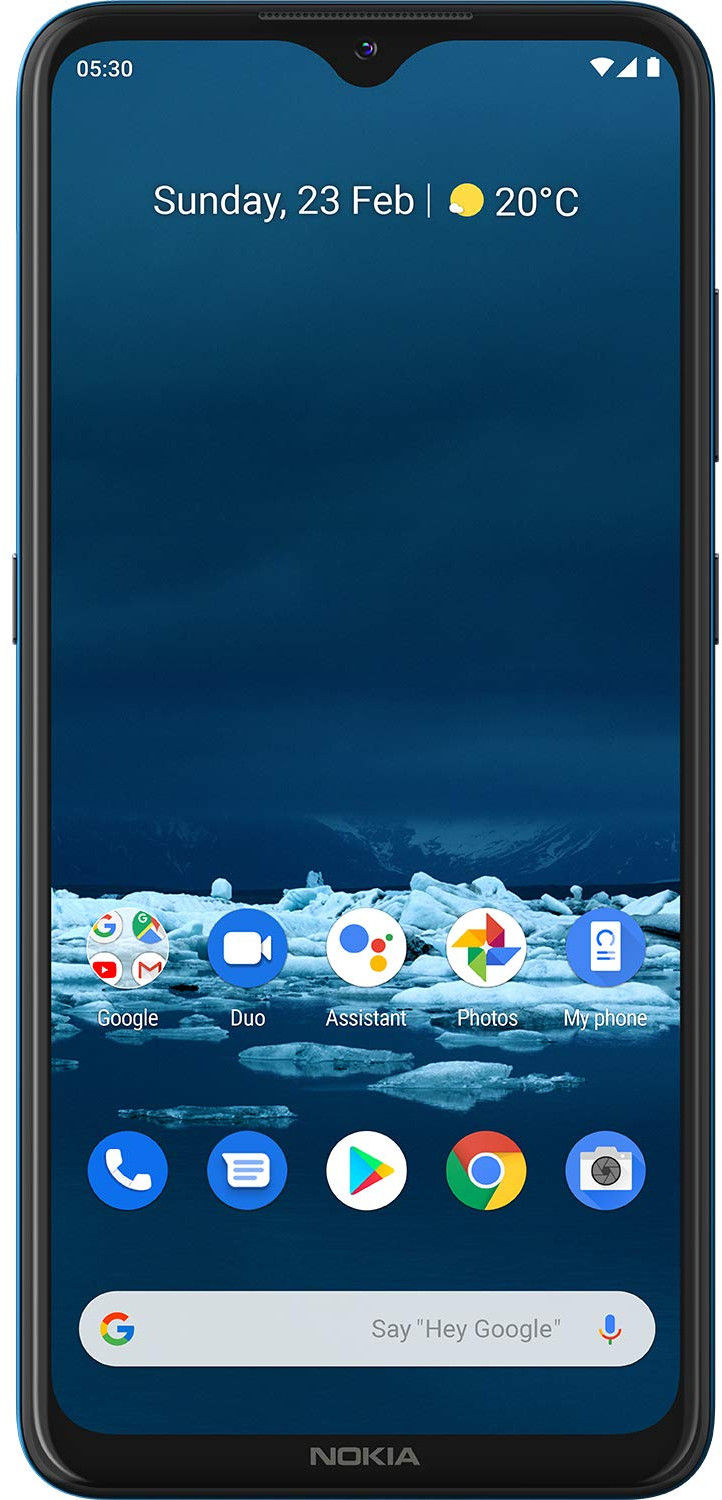The image showcases a black cell phone with a detailed and serene wallpaper against a dark navy blue background. The wallpaper features distant dark blue mountains capped with bright white snow and a foreground of dark blue water interspersed with large, thick chunks of ice. At the top of the screen, the date is displayed as "Sunday, 23rd FEB," followed by a small vertical line. Next to it, an icon of the sun with a tiny white cloud to its left signifies clear weather, accompanied by the temperature reading, "20°C."

Below the date and weather information, there are several app icons: Google, Duo, Assistant, Photos, and an app labeled "My Glow-In." Further down, a series of circular app icons are visible: a blue circle with a white telephone symbol, a blue circle with a white notebook symbol, a white circle featuring a colorful arrow (representing Google), the Google Chrome icon with a blue center and an outer ring in red, yellow, and green, and a blue circle with a camera symbol inside.

At the bottom of the screen is a long, open search bar. In light gray text, it prompts, "Say Hey Google," accompanied by a microphone icon to the right.